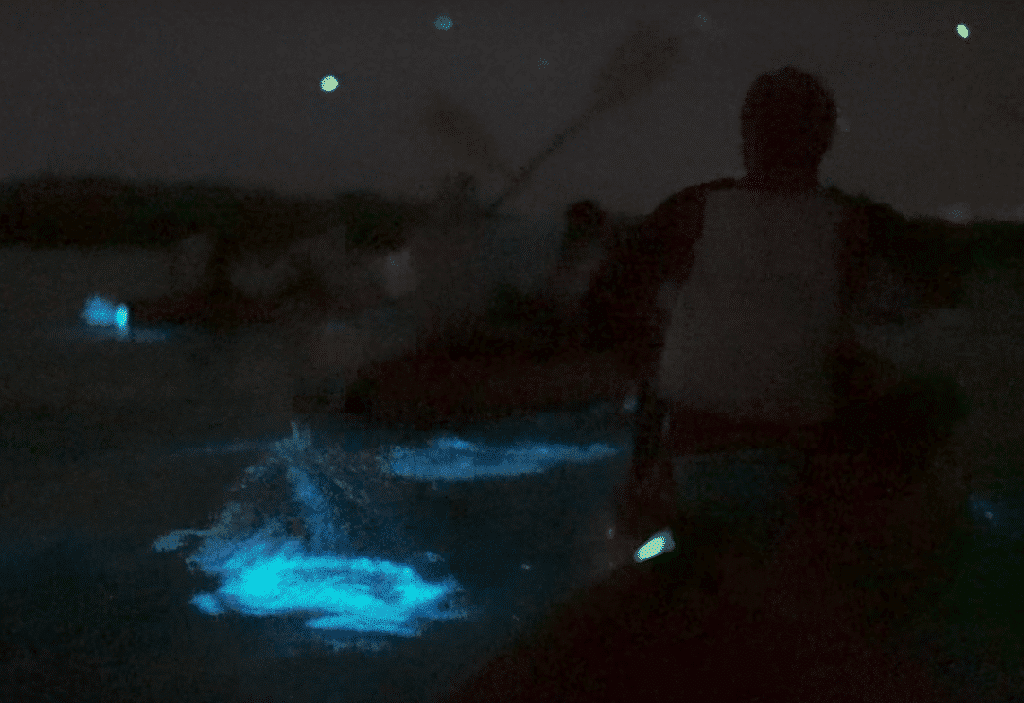In this blurry nighttime image, the scene captures the silhouette of a man in the immediate foreground, his back turned to us, wearing a tank top or wife beater and holding a flashlight. In the middle of the image, a cerulean-blue light highlights the water, which appears to be splashing, suggesting recent activity. This scene unfolds in or near a pool with a glowing blue hue, appearing as though someone or something has just leaped into the water. Situated on a body of water, the image depicts three kayaks: one on the far left, one in the middle, and one close to the right. The kayakers' raised oars are visible, and the glowing spots in the water beneath them illuminate the dark blue surface. Each kayaker seems to be wearing a white life vest. The distant background reveals faint lights on the horizon, either from streetlights, the moon, or possibly an airplane's trail, against a very dark sky sprinkled with a few stars.